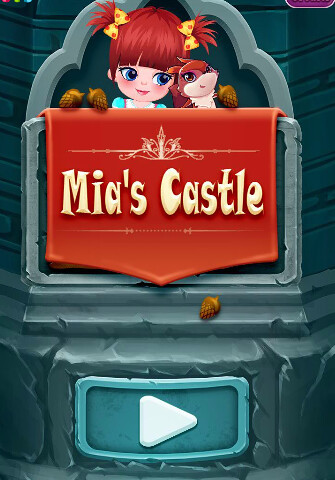"This vertical portrait-style image appears to be a colorful 3D rendering from a video game. It showcases a magnificent bluish-gray castle, intricate in detail, set against a vibrant backdrop. Towards the bottom of the image, there's a prominent play button, signified by a white triangle pointing to the right. Above the button, a crimson-red piece of fabric unfurls with 'Mia's Castle' emblazoned in bold yellow letters. At the very top, the focus shifts to an adorable character scene: a little girl with striking red hair adorned with yellow bows stands cheerfully beside a small, friendly-looking dinosaur. The whimsical, animated style of the image captures a sense of adventure and fantasy."